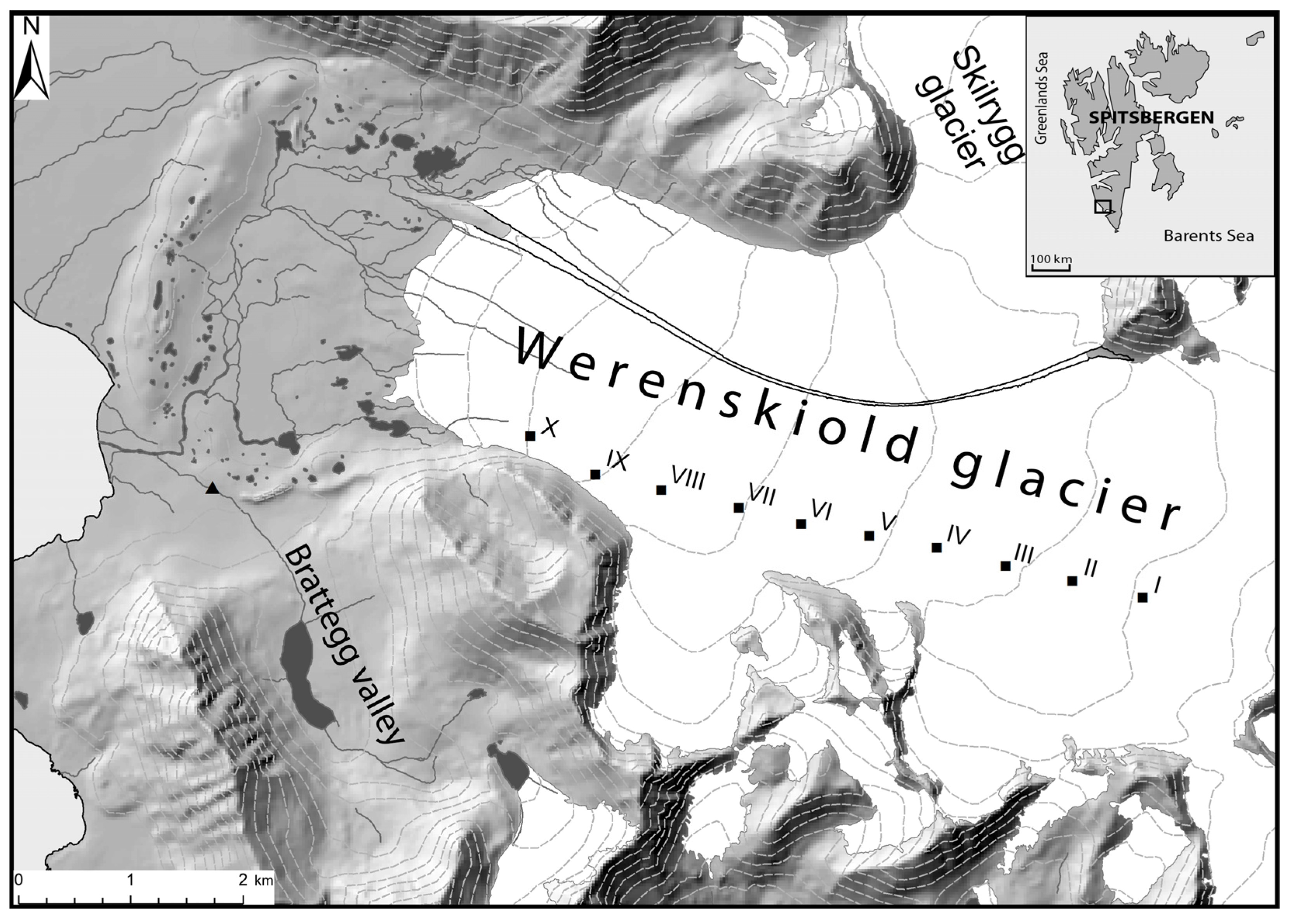This detailed topographical map illustrates the region around the Wernskold Glacier, prominently featured in the center-right portion of the map. The glacier is marked with contour lines and numbered guides using Roman numerals from I to X, indicating its elevation and structure. Adjacent to the Wernskold Glacier, on the left side of the map, lies the Brahek Valley, which appears in lighter shading compared to other regions. Positioned above the main glacier is the Skjelreg Glacier, adding further detail to the map's depiction of the terrain. In the top left corner, a symbol indicates the map's orientation as north-facing. A scale representing two kilometers can be found in the bottom left corner. Additionally, the top right corner features an inset map showing the broader geographical context, including Spitsbergen, the Barents Sea, and the Greenland Sea, with a 100-kilometer guide scale. The map uses various shades to differentiate between land elevations and potential bodies of water, emphasizing the diverse topographical features of this region.